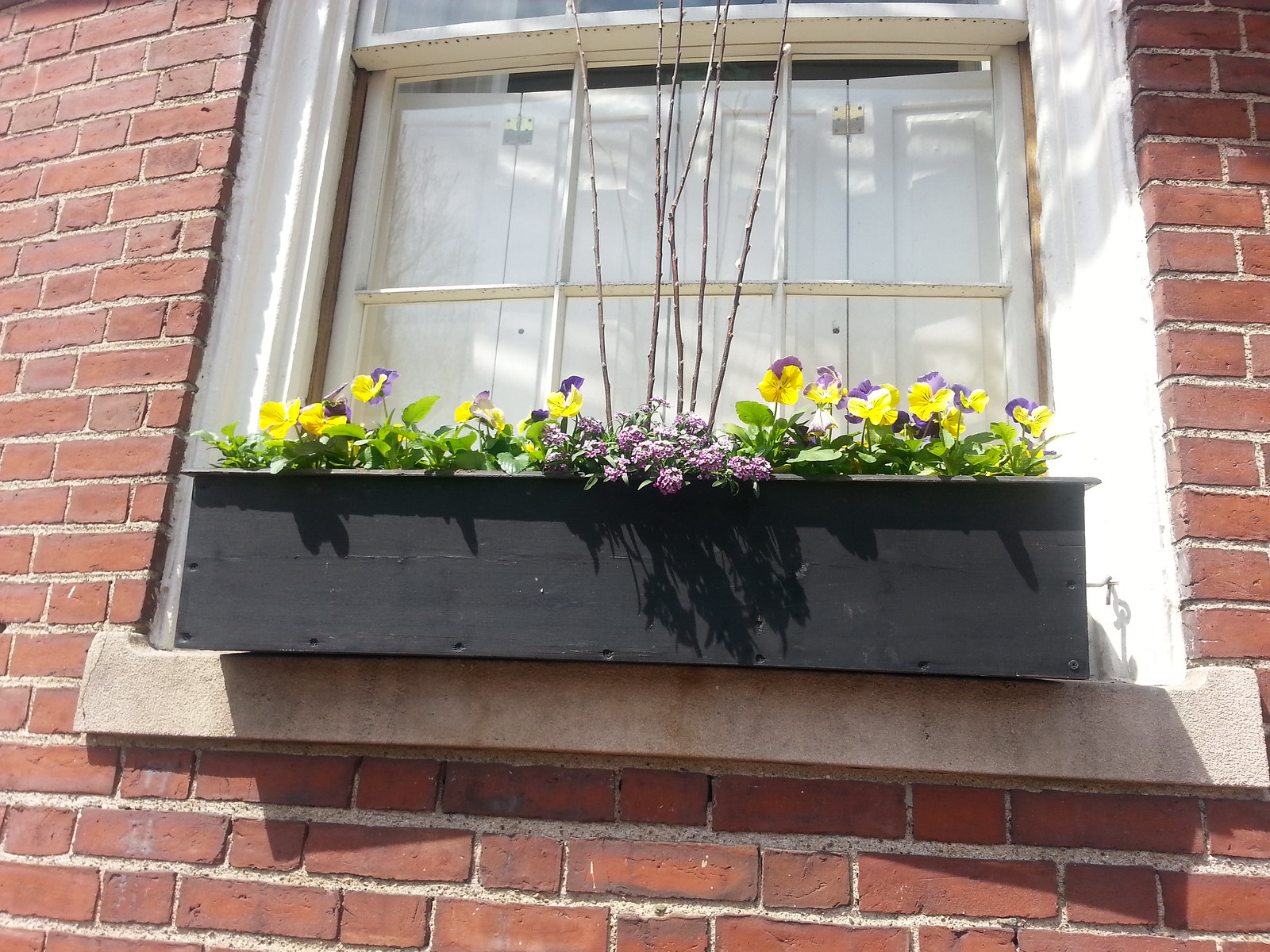In this outdoor daytime photograph, the focus is on a charming scene featuring a concrete gray ledge supporting a black window box filled with an array of vibrant flowers. The brick wall, composed of red bricks with white mortar, provides a rustic backdrop. Above the ledge, a window framed in white with six glass panes is flanked by white wooden shutters that obscure the interior.

The window box is bursting with color and life, showcasing purple and yellow violets alongside an assortment of other purple blooms. A rich tapestry of green leaves adds volume to the display, while five distinctive pussy willow stems emerge from the center, adding height and texture. The scene is bathed in sunlight, which casts soft shadows on both the window box and the wall, enhancing the textures and colors of the flowers and their surroundings.